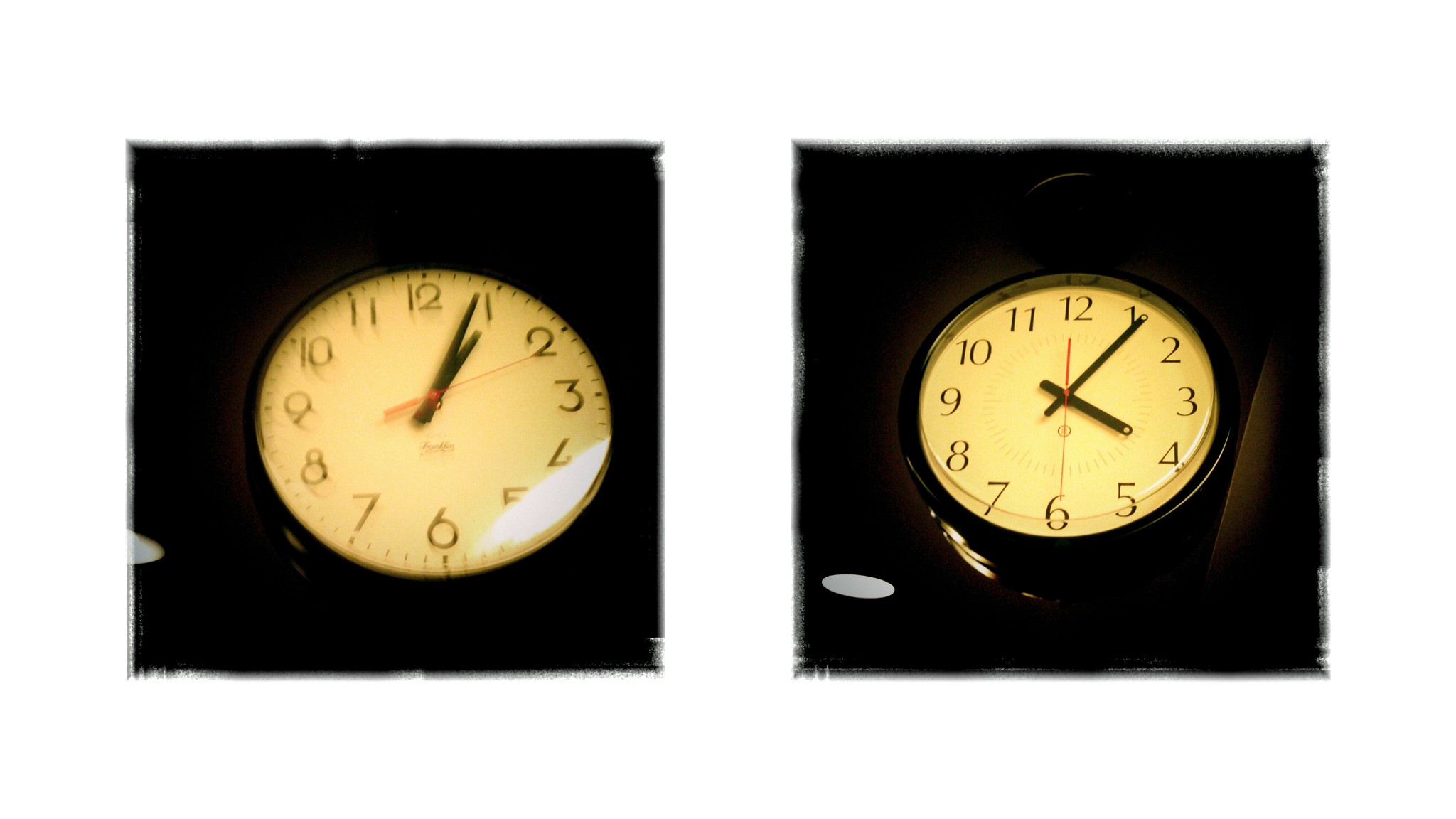The image comprises two contrasting square photographs, each featuring a distinct round wall clock. Both images share a consistent black background with subtly jagged edges—particularly noticeable in the top left and bottom right corners—and a faint gray border around them.

**Left Image:** 
This clock's face is white with classic black numerals encircling it. The time displayed is 1:04. The clock appears to be positioned flat against the background, enhancing the visibility of its simplistic design.

**Right Image:**
The second clock, displaying the time 4:06, is depicted with a black frame that contrasts sharply with its white face and black numerals. The seconds hand is precisely aligned with the 6, suggesting a moment frozen in time. This clock is oriented as though it is hanging from the ceiling, providing a more dynamic and focused view compared to its partner.